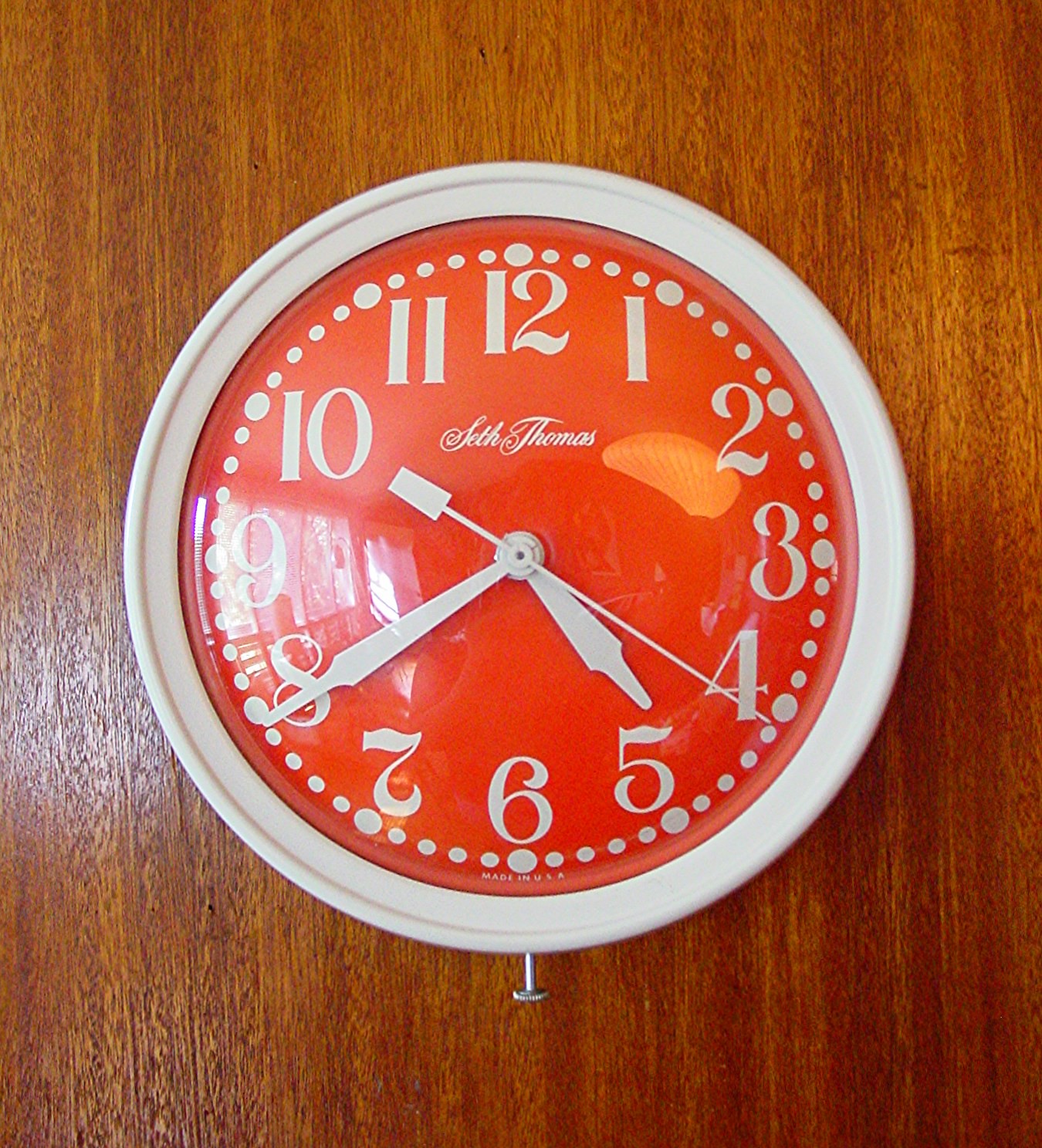This portrait-oriented photograph captures a visually striking clock mounted on a wall featuring medium brown wood paneling with vertical grain patterns. A subtle light highlights the left section of the wall, giving the paneling a slightly lighter, almost white hue in that area.

Central to the image is a prominent circular clock, occupying roughly 70% of the frame’s width, leaving about 15% of space on either side. The clock's frame is white, likely plastic, enclosing a vibrant orange face with a reddish undertone, reminiscent of vintage 1970s style. A reflective covering, possibly plastic or glass, protects the clock face and casts light reflections on its left side.

The clock face is marked by large, white standard numerals, with the 12 at the top and the six at the bottom, including each hour from 1 to 11. Between these numerals are smaller dots representing the minutes, grouped into four between each number. Larger dots are found adjacent to each numeral. Below the number ten, the brand name "Seth Thomas" is elegantly inscribed in white cursive.

The clock's hands are distinct in their design: the short and stout hour hand points just shy of the 5, the elongated minute hand almost touches the dot above the 8, indicating the time as 4:40. The thin, elongated second hand, balanced by a rectangular counterweight, hovers just past the 4 on the lower right.

Below the clock's center mechanism, a silver dial protrudes slightly, likely serving as the adjustment mechanism for setting the time, resembling a screw in appearance. This detailed and nostalgic depiction of the clock exudes a sense of retro charm combined with functional simplicity.